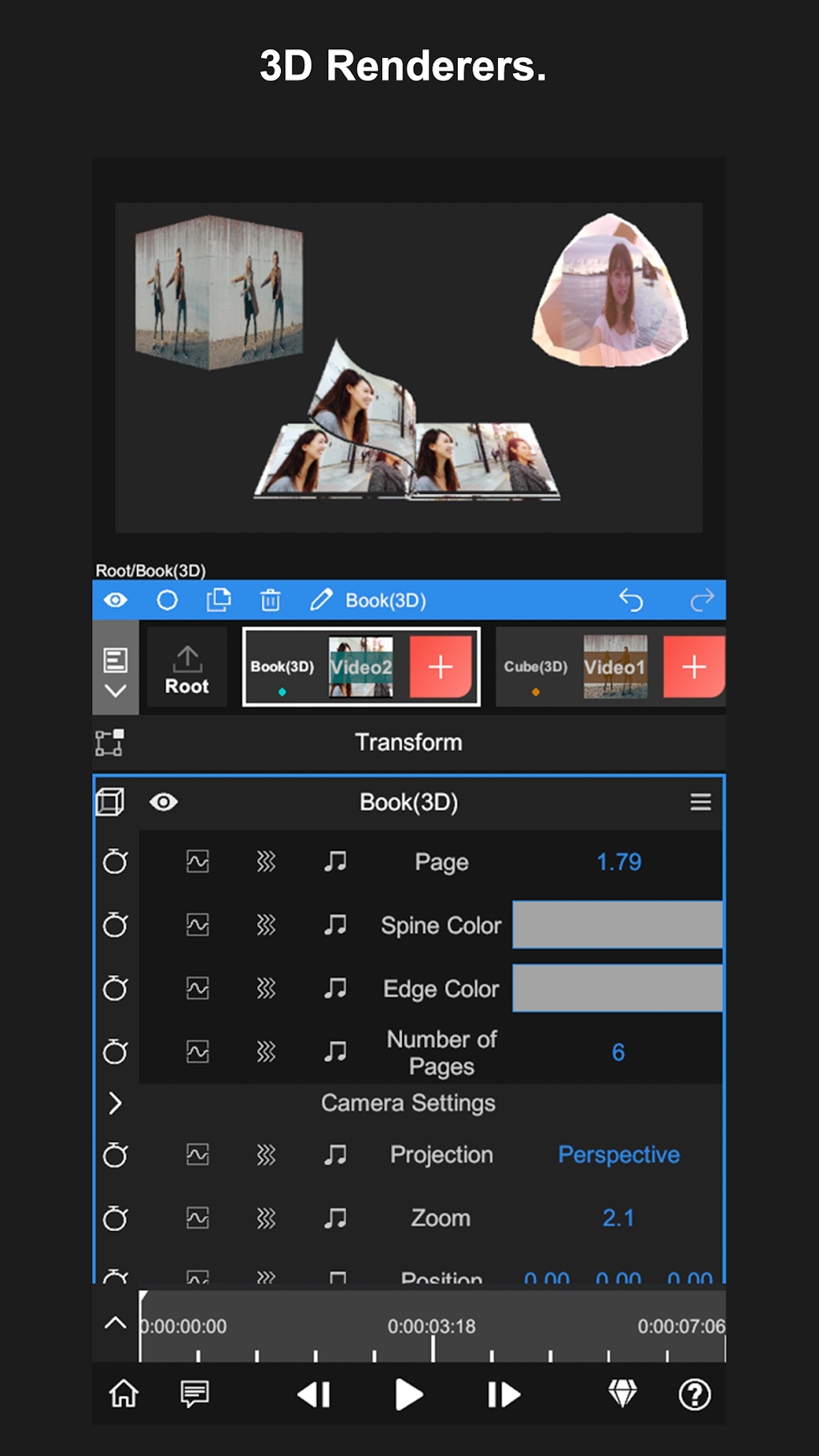This is an image depicting a screenshot from a mobile application. The application interface has a sleek black background, which serves as a contrast to the vivid content displayed. 

At the very top of the screen, in bold white letters, are the words "3D Renderers," clearly identifying the feature or section of the app. Directly beneath this title, there is a rectangular section on a gray background that contains a collection of three images. 

The first image within this collection features an illustration of an open book, displaying a detailed scene with two women. The second and third images, although partially visible, complete this trio of visuals presented on the gray backdrop.

Immediately below this assembly of three images, the app showcases another distinct image—this one illustrating the interface of a 3D book application. The app interface prominently includes a blue banner positioned at the top of the screen, which draws the viewer's attention. In the upper left corner of this blue banner, there is a small white icon depicting an eye, possibly indicating settings or a view mode.

Underneath the blue banner, in clear white text, the word "Transform" is displayed, hinting at a potential function or feature related to the 3D rendering capabilities of the app.